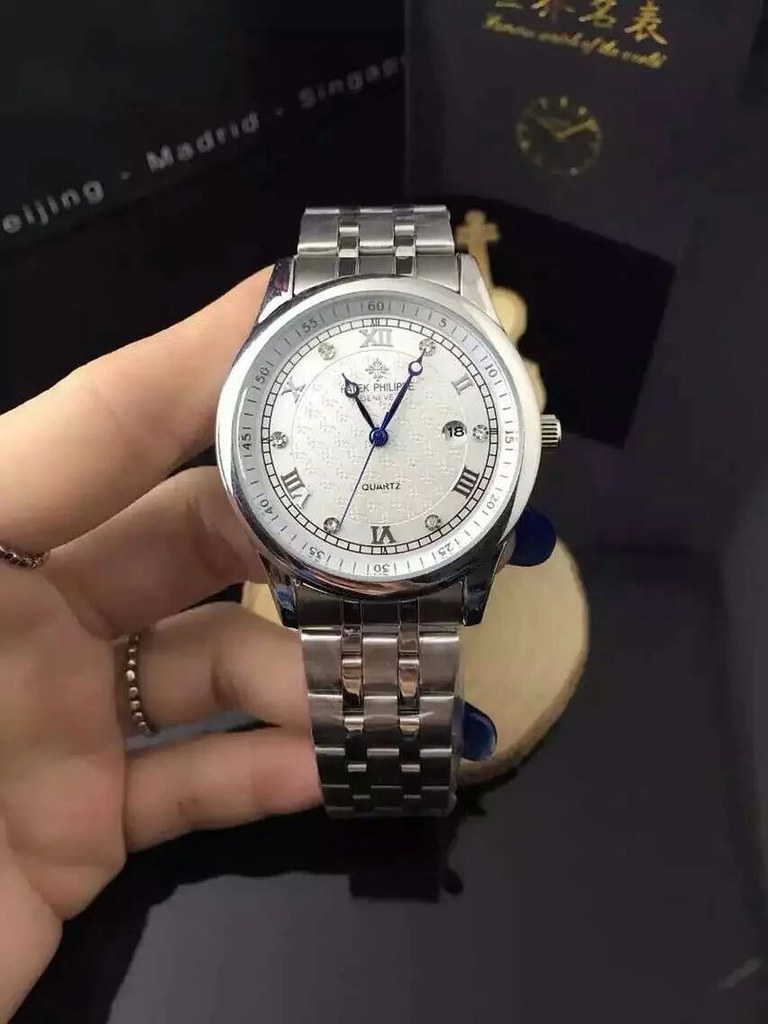The image portrays an elegant display of a silver wristwatch. The background is a deep black, providing a striking contrast to the watch's details. In the upper left-hand corner, gray lettering spells out names of major cities such as Beijing, Madrid, and Singapore, against the dark backdrop. 

A refined wooden stand holds the watch, resting on a black base that enhances the sophisticated presentation. A booklet, black with gold writing and adorned with a gold clock face, lies beneath the watch, adding to the luxurious aesthetic. 

Adding a personal touch to the scene, a woman's hand, adorned with several delicate rings, holds the timepiece. The watch features a classic design with Roman numerals encircling its face and elegant blue hour and minute hands. The subtle play of shadows accentuates the overall composition, highlighting the watch as the focal point.